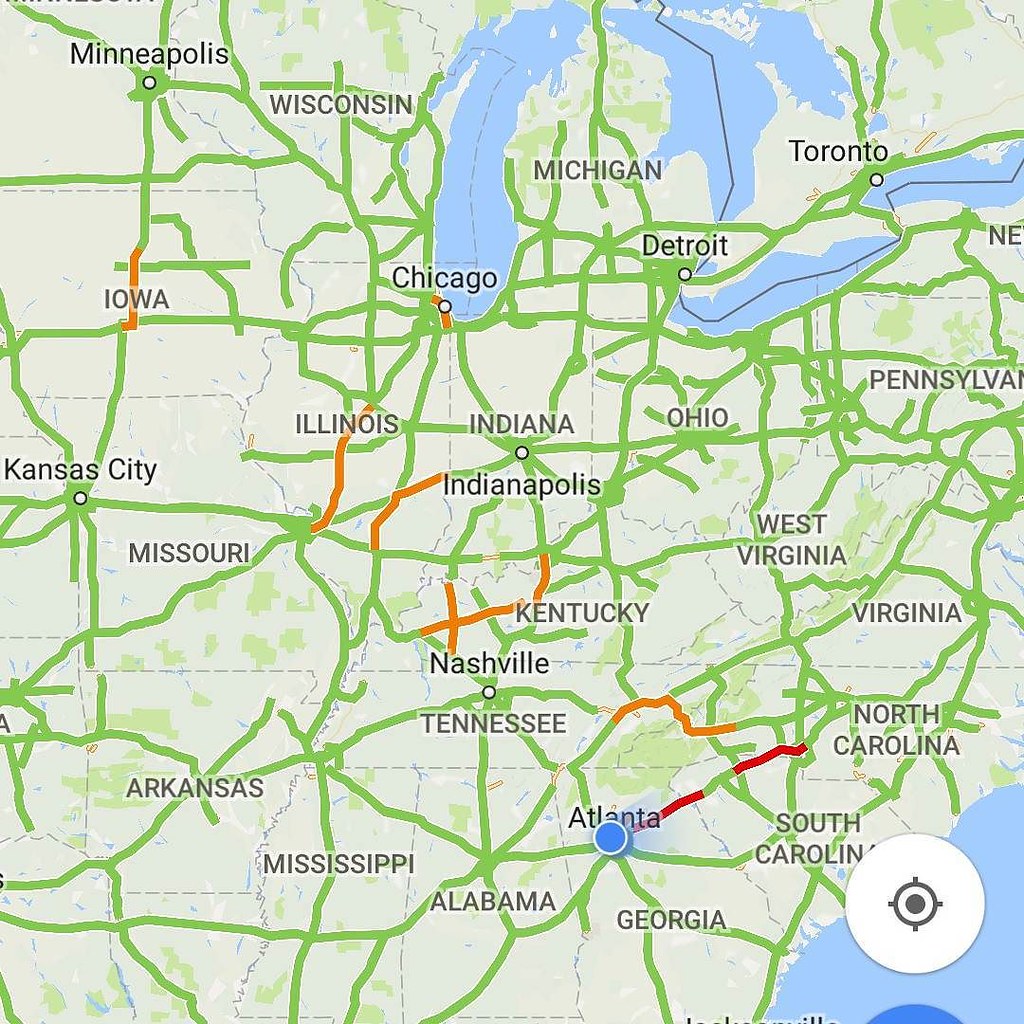This image is a screenshot from a map application, possibly Google Maps or Apple Maps, showcasing the eastern United States. The map extends from Kansas City on the far left to Pennsylvania on the far right. Major geographical features include the Great Lakes, illustrated in blue. Various lines indicate different types of routes and highways across the region. Green lines traverse states like Iowa, Illinois, and Kentucky, while orange lines are visible in the same areas, suggesting moderate traffic congestion. In the southern part of the map, including Atlanta and parts of North Carolina, red lines denote heavy traffic or road closures.

A prominent blue circular marker with a white border highlights Atlanta. In the bottom right corner, near South Carolina, there's a white circle containing a gray dot, likely a zoom control button. Additionally, part of another blue circle is visible in this corner, but its full purpose is unclear. Overall, the screenshot provides a detailed view of traffic conditions and major landmarks in the eastern United States.